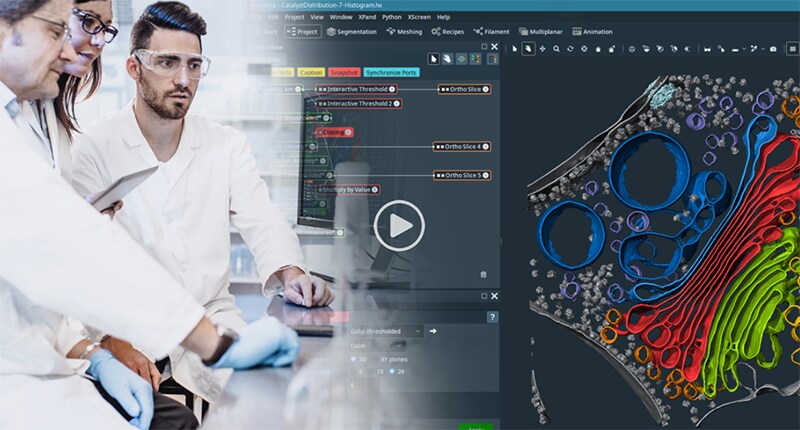The image appears to be a paused frame from a video, indicated by a yellow play button in the center. On the left side, three individuals—two men and one woman—are seated behind a desk in a lab-like environment. All three are dressed in white lab coats, with one man wearing goggles, the other man and the woman are wearing glasses. The older man, distinguishable by his blue gloves, is seated next to the woman with longer hair and glasses. They are all focused on a computer screen in front of them. 

The right side of the image displays what appears to be a detailed, colorful graphic that the group is examining on the computer. It resembles a microscope image of a cell, showcasing various vividly colored elements such as red, blue, and green bubbles, alongside long, strand-like structures. The segments are multi-colored, including hints of orange, purple, and gray against a dark background. Text at the top of the computer screen includes terms like "snapshot caption synchronized parts," although it's partially obscured. The array of colors and complex details suggest an intricate biological or scientific visualization.